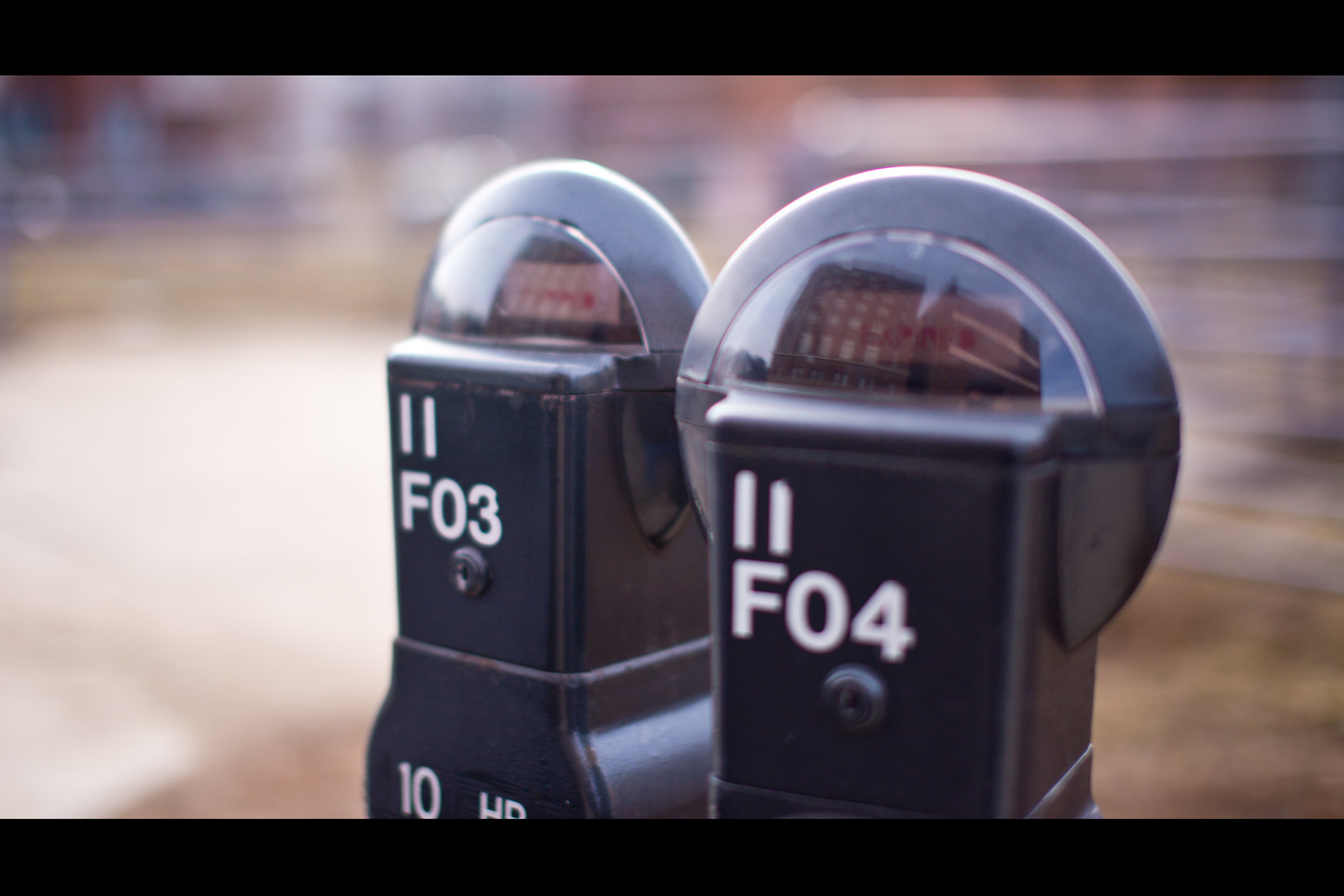This horizontally oriented, slightly blurry, color photograph—likely a screenshot with black bars at the top and bottom—features a close-up of two black parking meters standing side by side in the center of the frame. In bright daylight, the left meter displays the white lettering "11F03," followed by "10HR" beneath it. The right meter shows "11F04." Both meters possess a reflective glass surface at the top, mirroring the image of tall, industrial-looking buildings, possibly high-rise apartments, in front of them. The background is blurred with muted colors, indicating light and movement, including gray and brown splotches, and a hint of green grass, suggesting a nearby paved road or gravel driveway.